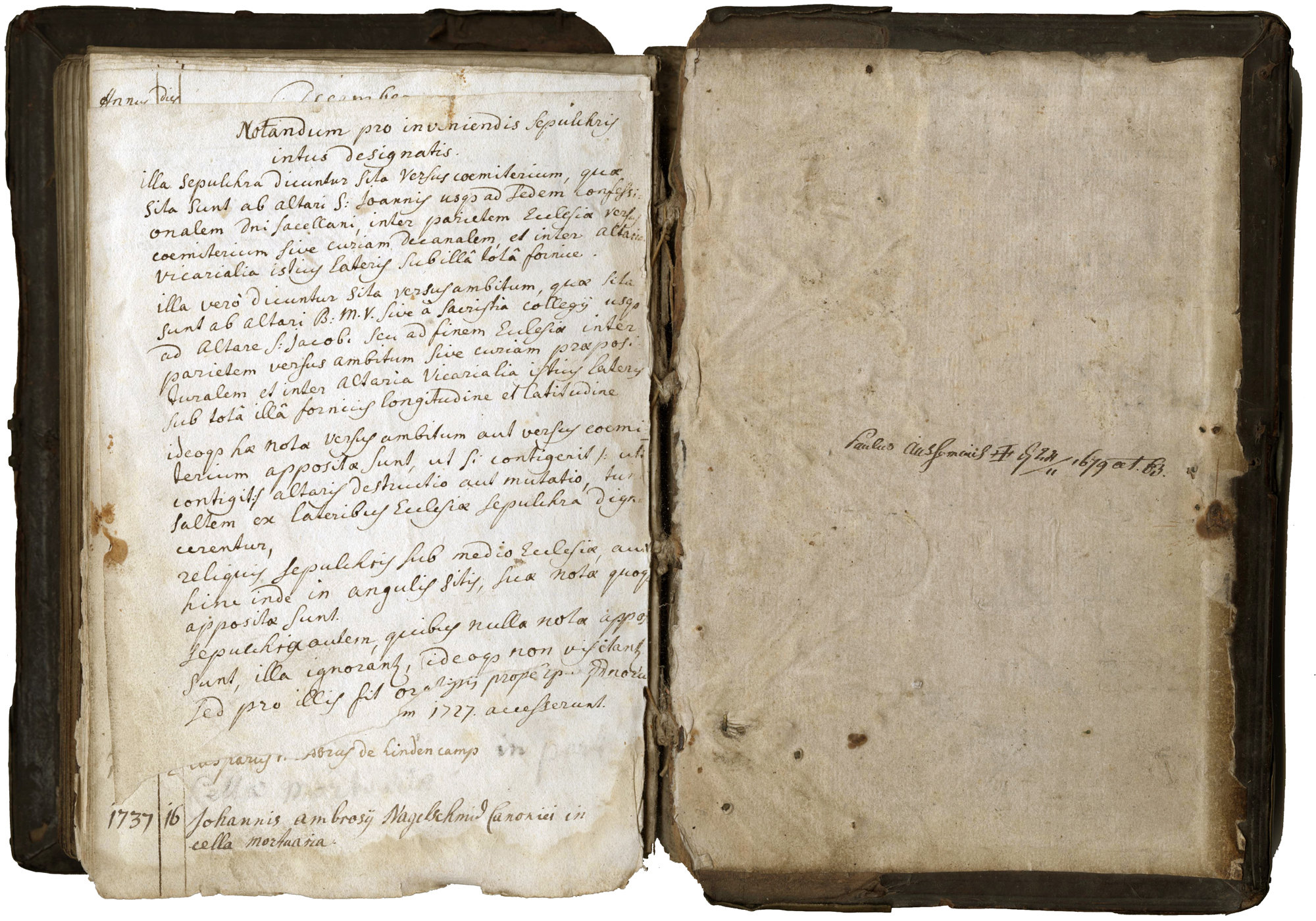The image depicts a photograph of a very old, tattered, and torn book. The book is open to a page, revealing its severely debilitated binding, with the spine looking rotted and held together by merely a thread. Both the brown or black cover and the edges of the pages are visibly worn out, ripped, and darkened, indicative of the book's advanced age. The pages themselves are fragile and thin, with a brownish-tan hue, showing signs of significant wear and tear, including spots and smudges.

On the left page, there is handwritten cursive writing, which is elegant and in calligraphy style, filling the entire surface. This writing appears to be in Latin, and at the very bottom of the page, the date "1737-16" is discernible, suggesting the book's origin from the 18th century. The text at the top of the left page is in a different language and is not legible. The right page features just a single line of writing, also in an unknown language, contributing to the mysterious and ancient aura of the book. The meticulous manuscript and the journal-like appearance suggest it could have been a personal journal or military log from that era, its lines varying between straight and slightly diagonal. This venerable volume stands as a testament to its historical value and antiquity.